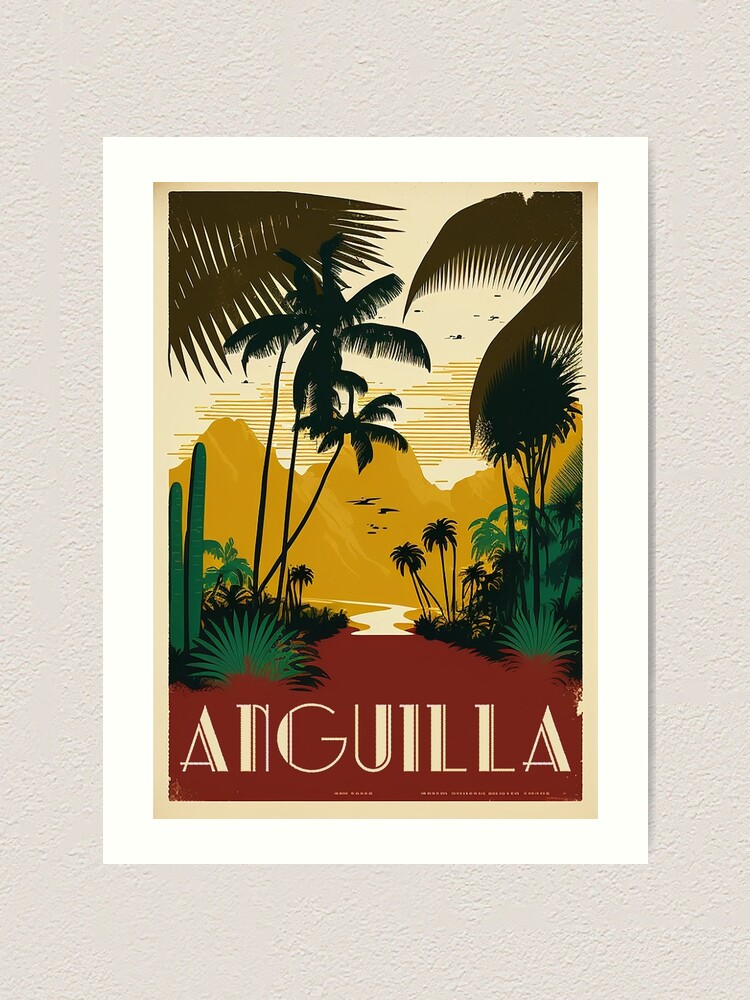The image showcases a vividly colored poster portraying a tropical scene, mounted on a textured white stucco wall. The poster itself has a white border surrounding a cream background, forming a square frame. The illustration within features a diverse palette, creating a striking and detailed depiction of a tropical landscape. 

In the foreground, green cacti and ferns flank the sides, while black palm trees and additional green foliage extend toward a central white, wavy creek. This creek meets a red-clay colored base, adding depth to the perspective. Further into the background, the vegetation darkens, transitioning into a yellow ochre mountain range set against a white to beige sky with yellow streaks, possibly representing clouds. Some birds are faintly visible in the sky.

Dingy brown-green palm tree leaves hang from the top corners of the image, contributing to the dense tropical ambiance. Below the scene, the text "Anguilla" is prominently displayed in a cream Art Deco font, reinforcing the tropical and inviting nature of the location depicted. The overall image is brightly illuminated, with meticulous detail and clarity reflecting a moment in a lush, tropical environment.